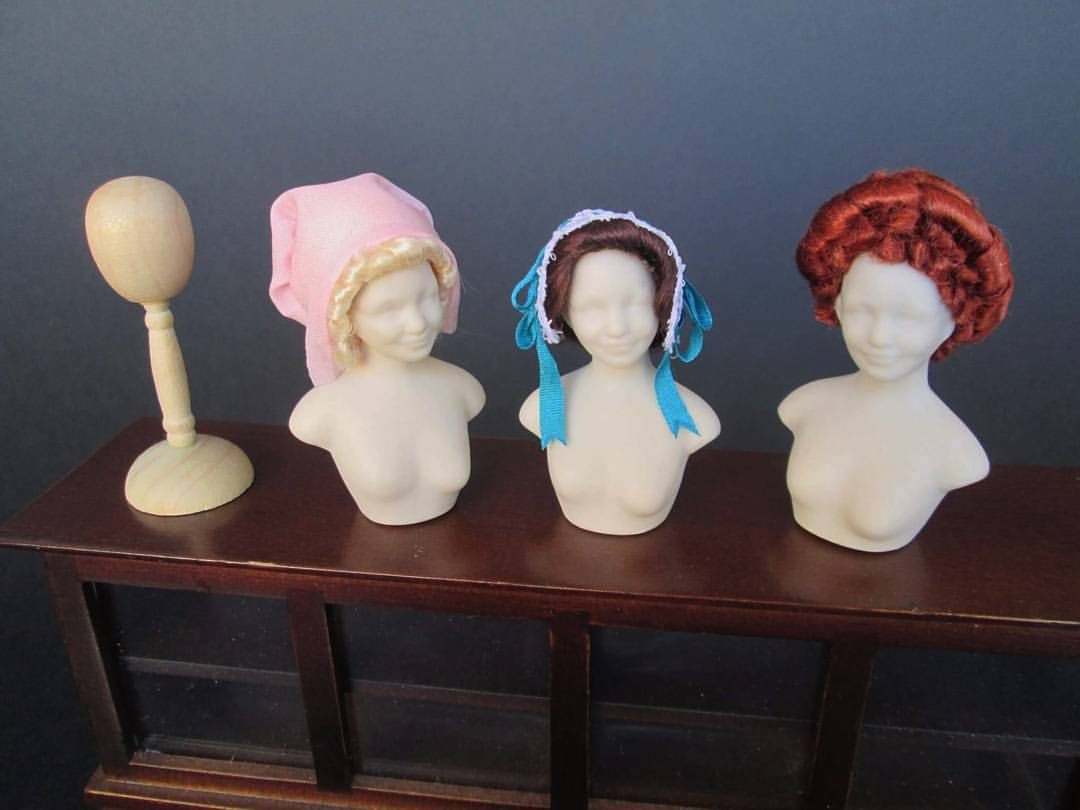In this photograph, we see four upper torso mannequins arranged on a dark red to dark brown wooden buffet table with glass shelving at the bottom and a sleek gray-blue wall in the background. The first mannequin on the far left has a distinctive wooden oval head mounted on a long base with a flat bottom and gently curved top; it lacks any facial features or a wig. The next three mannequins are torso busts of women, ending under the rib cage, with no arms but featuring shoulders and smiling faces with detailed facial features, though their eyes and eyebrows are left blank. The second mannequin sports a blonde wig topped with a pink sheath headpiece. The third mannequin showcases brown hair adorned with a blue and white bonnet. The fourth mannequin has a bright red curly updo reminiscent of 18th-century hairstyles, with no additional headpiece.